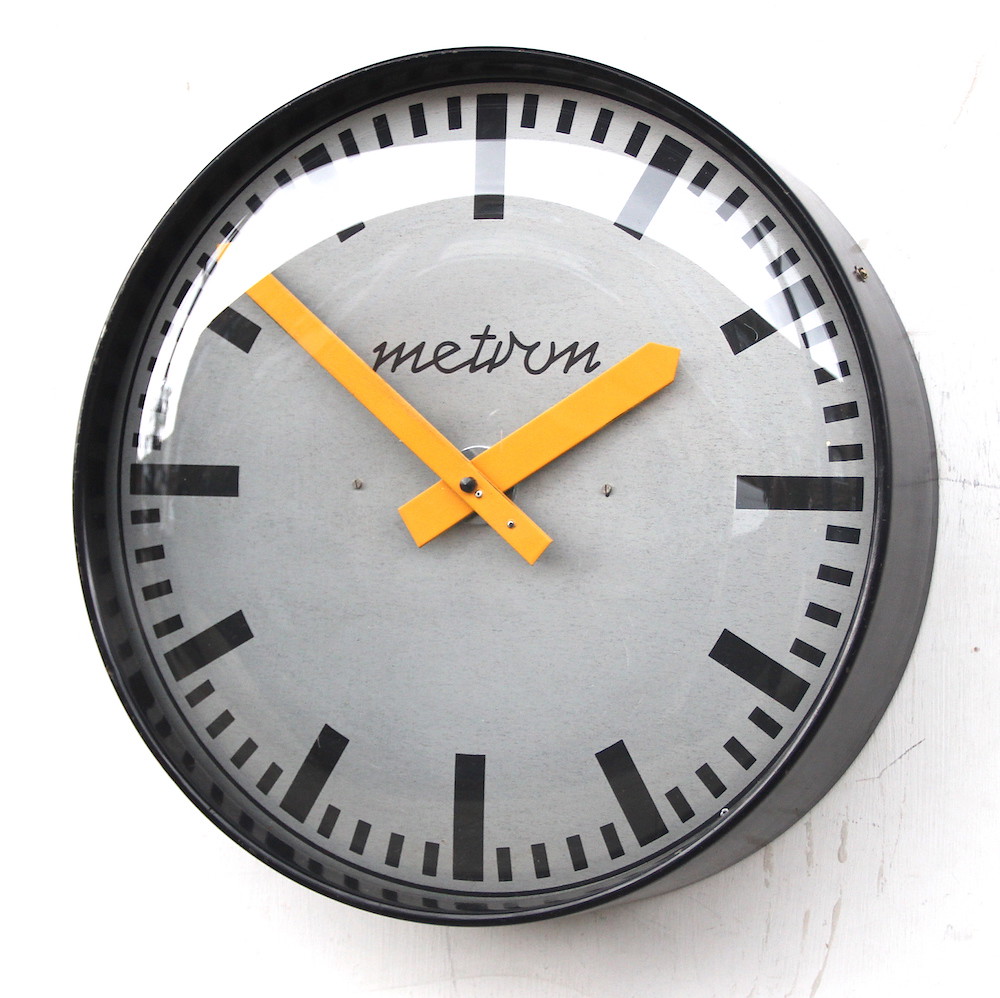The image features a centrally positioned wall clock with a black plastic frame against a white background. The clock face, protected by a glass cover that reflects light from the upper left, consists of a gray layer adorned with thick black hour markers and thin black minute markers. Around it, a subtle shadow falls to the right, suggesting the light source's position. The clock's hands—long and thin for the minute and second, and short and thick for the hour—are orange in color, with the hands indicating a time close to 1:51. Above the center of the clock face, the brand name "METIRM" is inscribed in a cursive-like font, though the 'I' appears somewhat unclear.